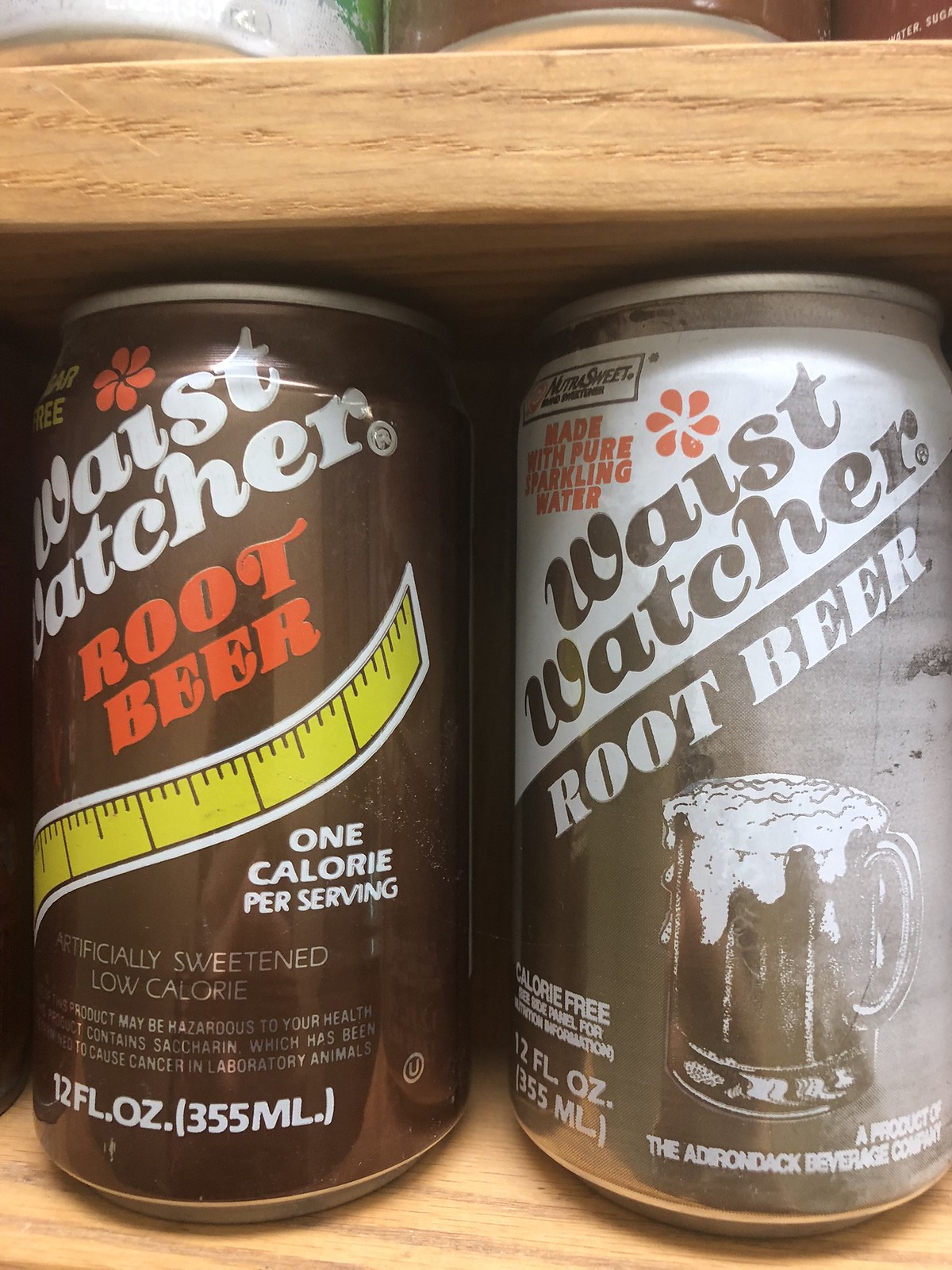The image depicts two cans of root beer placed side by side. 

The can on the left is from the brand "Waste Watches." It features a brown design with a clipart image of a measuring tape, signaling its low-calorie content. The label reads "root beer" and emphasizes its health-conscious appeal with phrases like "artificially sweetened," "low calories," and "one calorie per serving." The can holds 12 fluid ounces (355 milliliters). 

The can on the right is designed in grey and white tones and highlights its use of "pure sparkling water." It also bears the label "root beer," but opts for a different aesthetic with a large, overflowing pint glass illustration. This can is marked "calorie free" and, like its counterpart, contains 12 fluid ounces (355 milliliters). The stark contrast in design between the two cans highlights the different marketing appeals—one focusing on low calories and the other on the purity of ingredients.